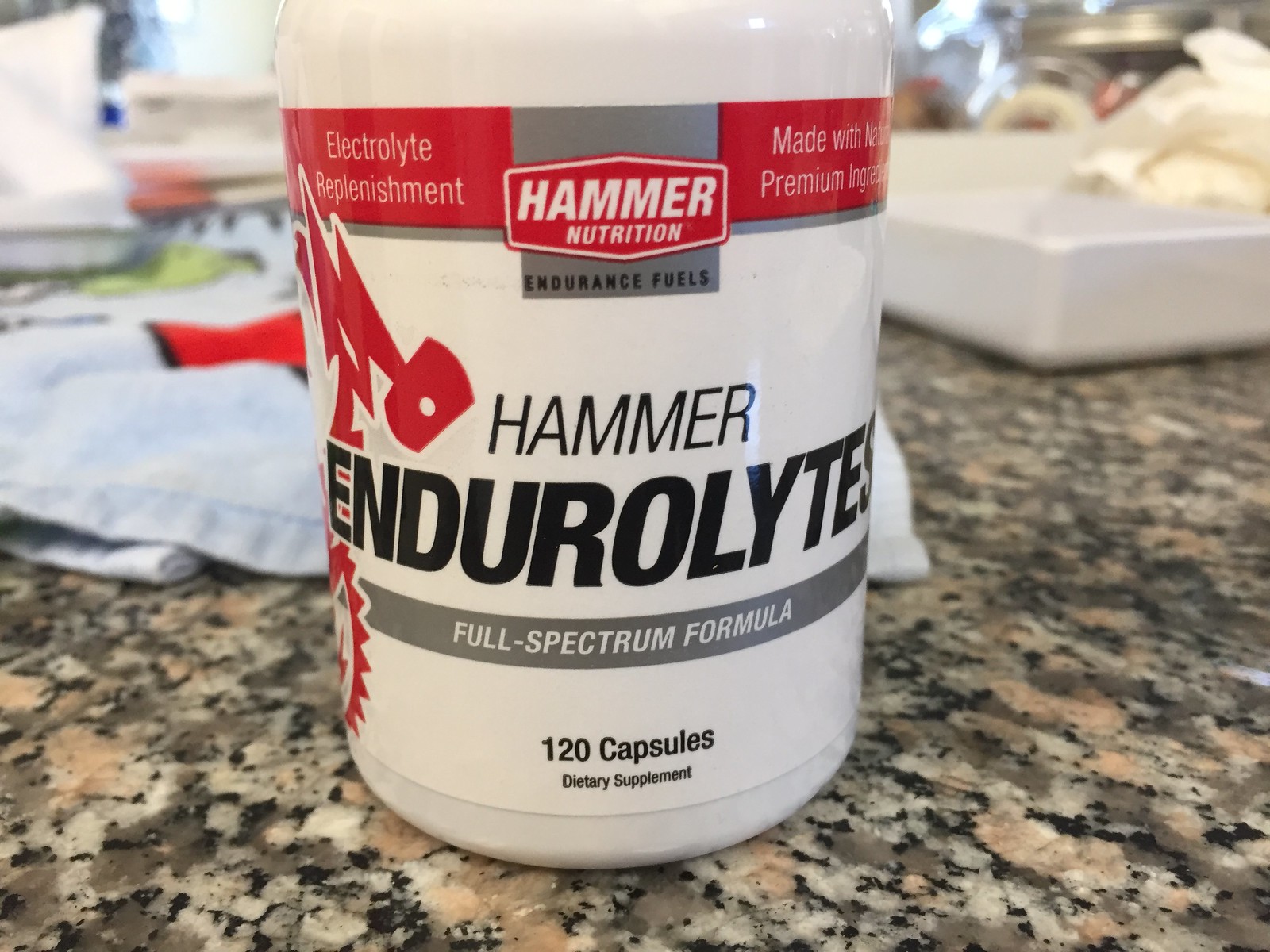The image features a large, clearly white plastic jar containing a white powder, though the edges of the jar appear translucent due to light reflection. The jar is prominently labeled with a red and white design, coupled with black and white text. The label reads "Electrolyte Replenishment" and "Hammer Nutrition" and also mentions "Endurance Fuels," "Hammer Electrolytes," and "Full Spectrum Formula." It specifies that the jar contains 120 capsules of a dietary supplement. The jar rests on a stone countertop that is marbled with browns, beiges, cream colors, and blacks. In the background, a variety of objects are visible, including a blue towel with red and green accents and a white tray. Additional indistinct, mostly white and silver objects are also present in the background.